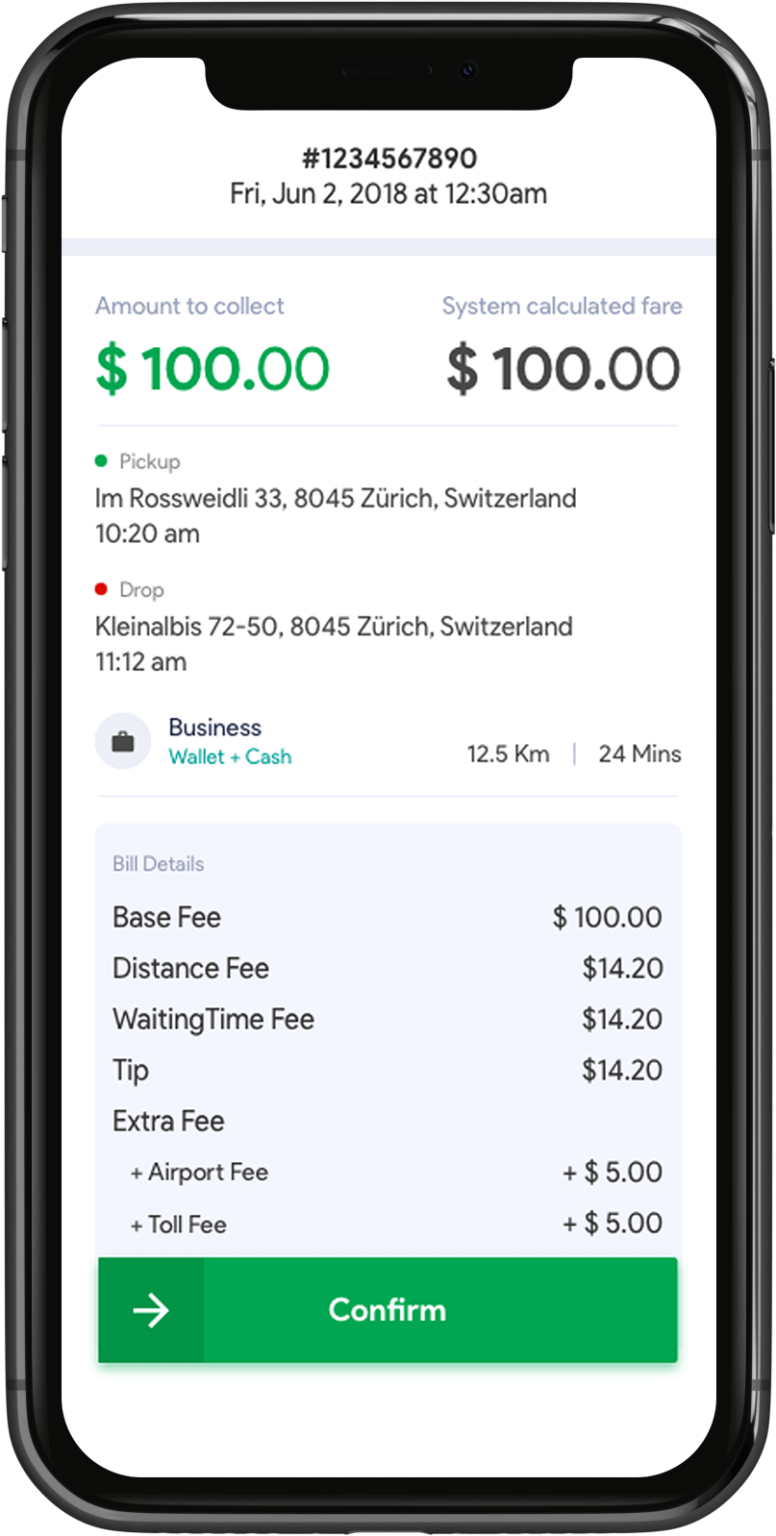In this image, we see a smartphone displaying a transaction screen. At the bottom of the screen, there is a green rectangle labeled "Confirm," accompanied by a left-facing arrow. Above this are detailed sections: a dark grey segment labeled "Bill Details," which itemizes charges such as base fee, distance fee, waiting time fee, tip, extra fee for the airport fee, and toll fee. Above the bill details, there are fields displaying the pickup and drop-off addresses. At the very top of the screen, an order number and date, "Friday, June 2nd, 2018 at 12:30 AM," are shown. The screen also indicates an "Amount to Collect" of $100 and a "System Calculated Fare" of $100 on the right side. The outer frame of the phone is visible, featuring the volume buttons on the left side. The background behind the phone is a plain white, drawing full attention to the details on the screen.